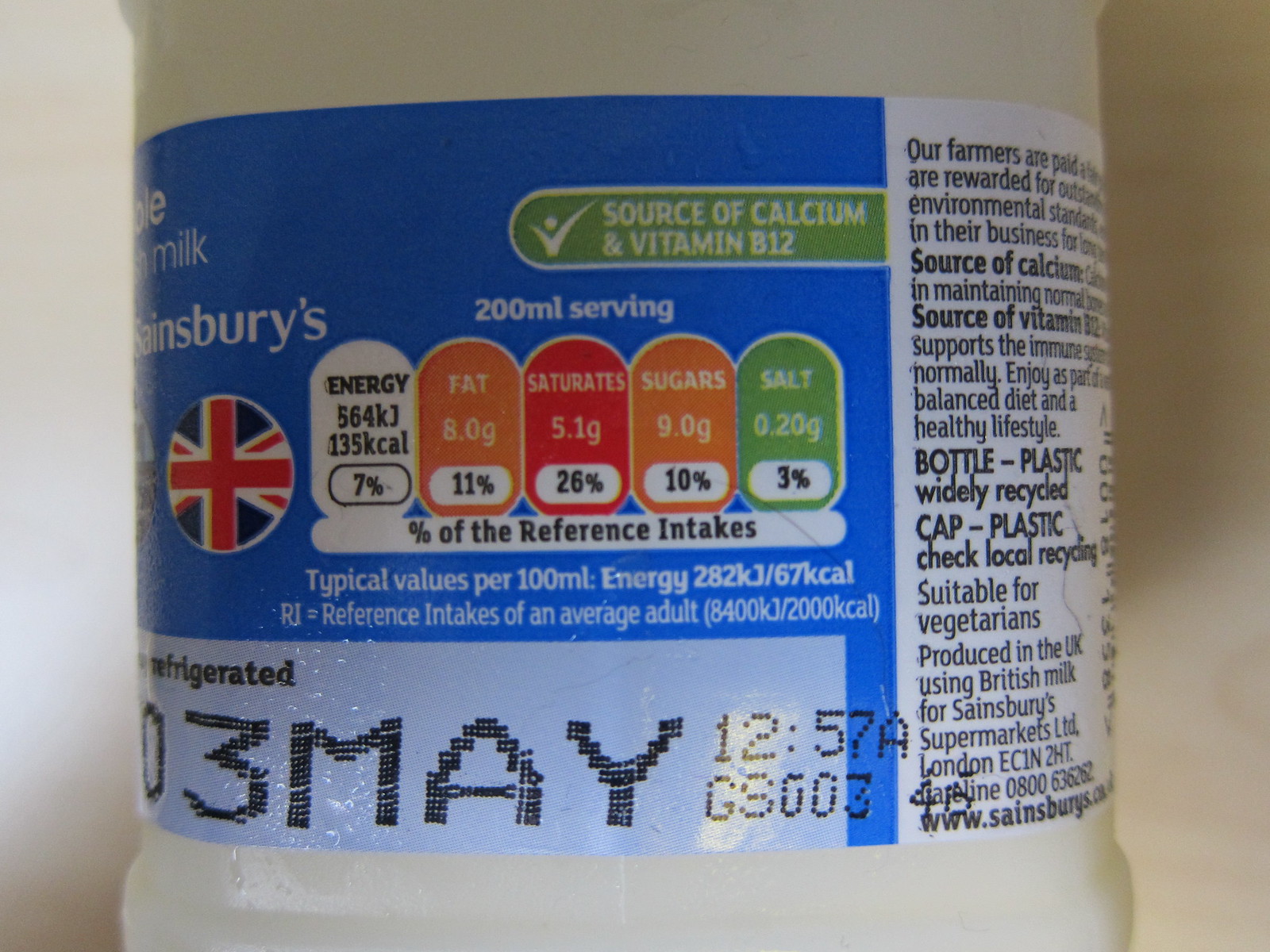This photograph captures a close-up of a plastic bottle, likely containing milk or a similar beverage. The bottle itself is white, and prominently displays a detailed label that combines shades of dark blue, light blue, and white. At the top left of the label, the background is dark blue, containing essential product information, including "Source of calcium and vitamin B12." Toward the middle and bottom left, the label shifts to light blue, where the expiration or manufacturing date "3 May 1257" is printed. The white section of the label is packed with text in black letters, providing additional details and instructions, such as the directive to "Keep refrigerated." Notably, there is a British flag symbol enclosed in a circle towards the middle of the label, signifying the product's origin or standard. Below this, the label lists nutritional facts in colorful ovals, detailing the amounts of energy, fat, saturates, sugars, and salt per 200 ml serving, highlighted by specific percentages for daily intake references. The overall label design organizes the nutritional and product information into easily distinguishable sections, providing a comprehensive overview at a glance.